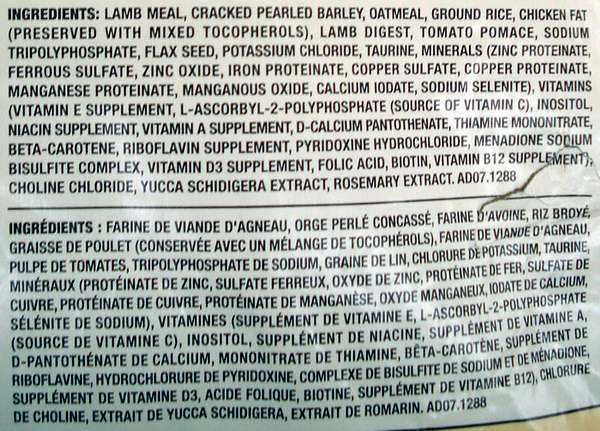This image captures the detailed ingredient label of a pet food product, likely for dogs or cats, written in both English and French on a wrinkled, white background. The top part of the label clearly lists the ingredients, starting with lamb meal, cracked pearled barley, oatmeal, and ground rice. Additional ingredients include chicken fat preserved with mixed tocopherols, lamb digest, tomato pomace, sodium tripolyphosphate, flaxseed, potassium chloride, and taurine. The list continues with an extensive array of minerals and vitamins such as zinc proteinate, ferrous sulfate, zinc oxide, iron proteinate, copper sulfate, copper proteinate, manganese proteinate, manganese oxide, calcium iodate, sodium selenite, vitamin E supplement, L-ascorbyl-2-phosphate (a source of vitamin C), inositol, niacin supplement, vitamin A supplement, D-calcium pantothenate, thiamine mononitrate, beta carotene, riboflavin supplement, pyridoxine hydrochloride, menadione sodium bisulfite complex, vitamin D3 supplement, folic acid, biotin, vitamin B12 supplement, and choline chloride. The label also notes the inclusion of yucca schidigera extract and rosemary extract. Beneath the English text, the ingredients are meticulously translated into French. The label appears slightly ripped at the right edge, emphasizing its worn condition. This rich and comprehensive list underscores the premium quality of the pet food, making it suitable for discerning pet owners seeking high-quality nutrition for their animals.